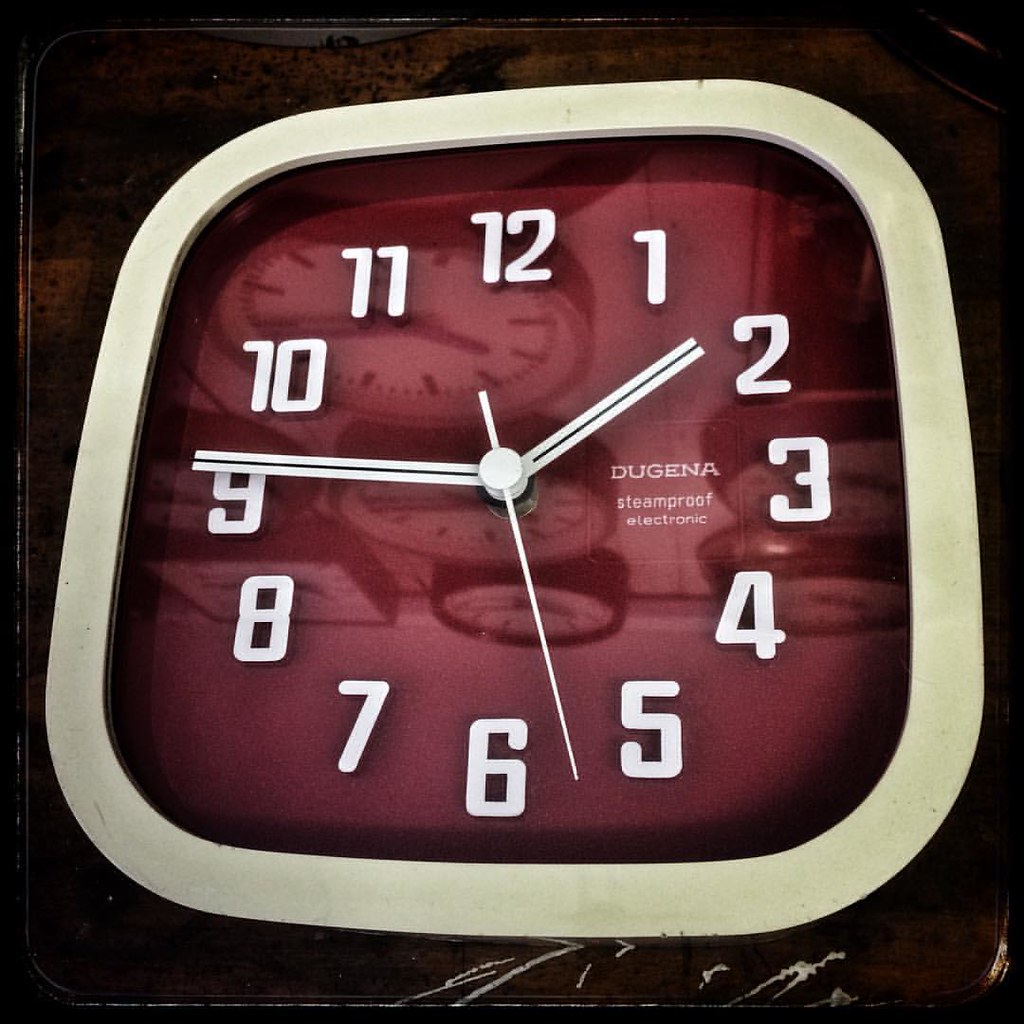The photograph captures a centrally positioned, retro-style analog clock with a distinct 70s era aesthetic. The clock features a rounded square frame with a beige or off-white outer edge and a dark wooden trim that shows some scratches, particularly on the lower part. The clock face is a striking red, with conventional numeric numbering from 1 to 12 in white, making it easy to read. The white hour and minute hands are thicker, contrasting with the thin second hand, and all are clearly visible against the red background. 

Notably, the clock displays white lettering that reads "Dugena Steam Proof Electronic." The time appears to read a quarter to 2 o'clock. Additionally, the red clock face reflects several other clocks—at least seven or eight—creating the illusion of little images within it. This reflective detail, coupled with the vibrant red background and clean white text and hands, highlights the clock's vintage charm while ensuring its functional elegance remains clear.